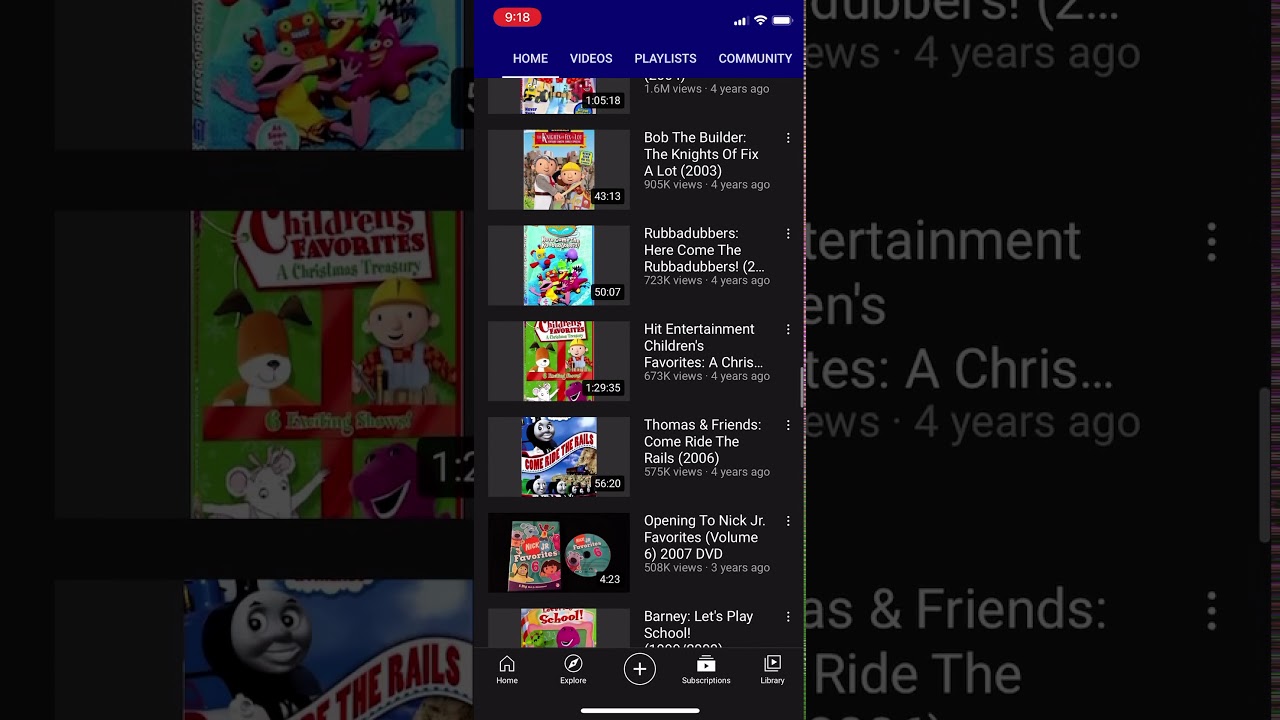A screenshot predominantly features a black desktop background. At the center, there's an embossed area resembling a mobile app interface. At the top left of this interface, the time is displayed as 9:18. The cellular signal is indicated as three out of four bars, Wi-Fi connectivity shows full strength with three out of three bars, and the battery is charged to either 92% or 95%.

Below the status indicators, four tabs can be seen: Home, Videos, Playlists, and Community. The Home tab is underlined, indicating it is the currently selected tab. 

Underneath the tabs, there is a list of video entries. The first entry is titled "Bob the Builder, the Knights of Fix-A-Lot (2003)." This video has 905,000 views and was uploaded four years ago. It has a duration of 43 minutes and 13 seconds.

The second video listed is "Rub-A-Dubbers: Here Come the Rub-A-Dubbers." It has garnered 723,000 views over the past four years and has a runtime of 50 minutes and 7 seconds.

The third video is titled "Hit Entertainment Children's Favorites: A Christmas Favorite." It has received 673,000 views from four years ago and lasts for 1 hour, 29 minutes, and 35 seconds.